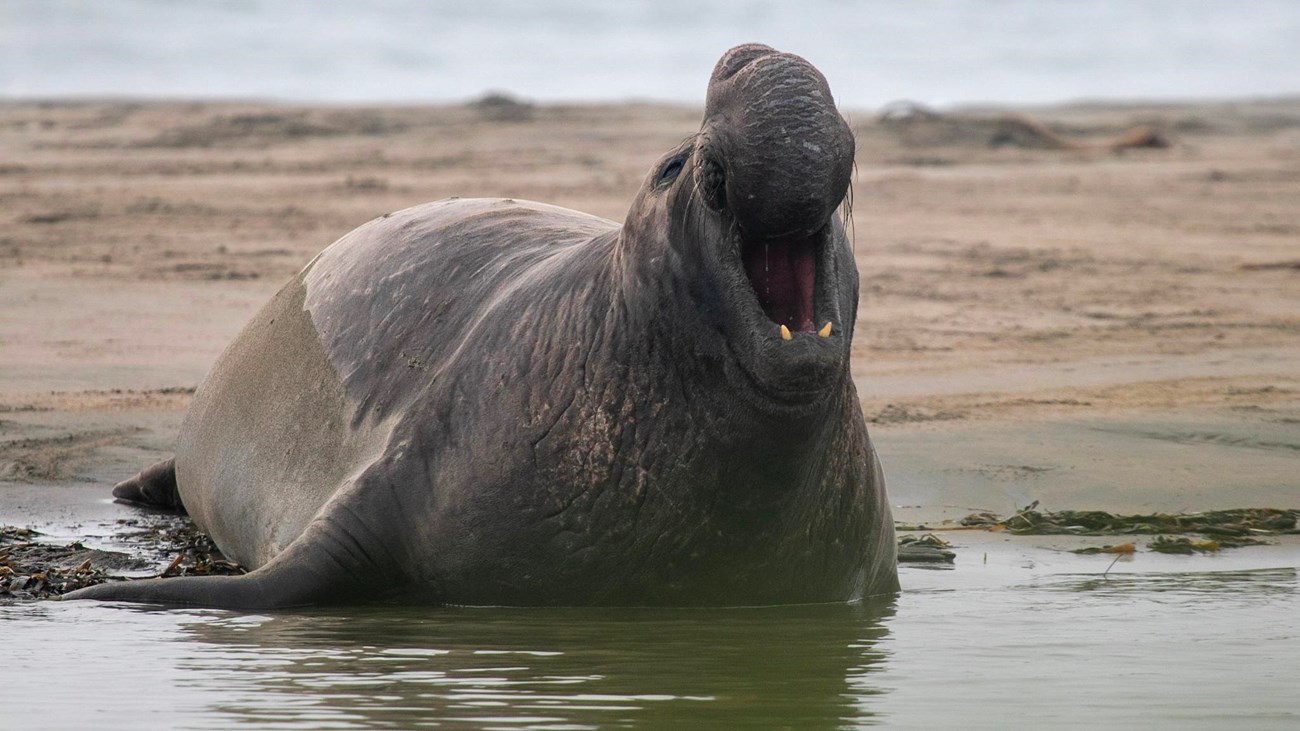This is a horizontally aligned rectangular image capturing a large marine animal, likely a walrus, positioned partially in shallow, rippling water with its rear end resting on wet tan-colored sand. The creature's substantial, flabby body varies in texture and coloration, with the back end appearing smoother and brown while the rest of its body shows darker brown and gray hues. Its head is lifted, mouth wide open, revealing small, yellowish teeth on its lower jaw, but there are no visible tusks. The snout is especially prominent. The cloudy sky, displaying shades of gray and white, forms the backdrop of this coastal scene. The setting suggests the animal might be vocalizing or barking as it wades into the water, which appears brown and slightly muddy. The photograph, taken during daytime, focuses entirely on this sizeable walrus in its natural seaside habitat, devoid of any textual elements or borders.